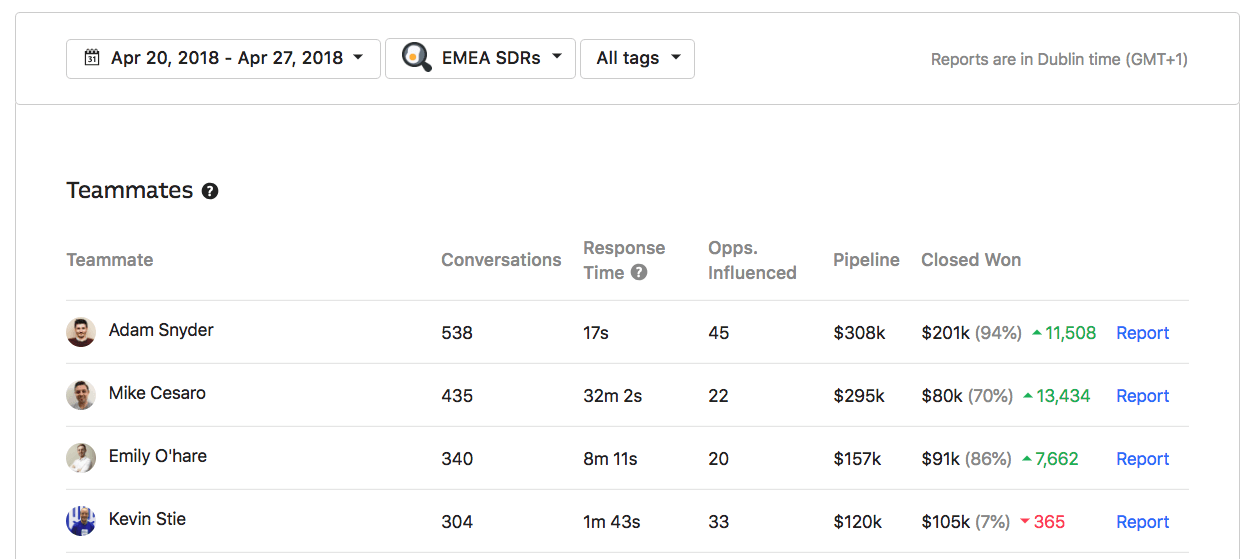This image, set against a white background, features a structured interface with several key elements organized from the upper left corner. 

**Top Section:**
1. **Date Selector:** "April 20th, 2018 through April 27th, 2018" displayed with a pull-down menu, accompanied by a calendar icon on the left.
2. **EMEA SDRs:** To the right of the date selector, a box labeled "EMEA SDRs" is present, with an icon of a magnifying glass and a pull-down menu.
3. **Tags Filter:** Another box labeled "All Tags" is situated further right, also with a pull-down menu.

**Time Zone Information:**
- A note indicates that the reports are in Dublin Time (GMT+1).

**Main Section:**
- Below these filters is a detailed list of teammates and their respective performance metrics. The details for each teammate are as follows:

1. **Adam:**
   - Conversations: 538
   - Average Response Time: 17 seconds
   - Ops Influenced: 45
   - Pipeline Value: $308K
   - Closed Deals Value: $201K

2. **Mike Cesaro:**
   - Conversations: 435
   - Average Response Time: 32 minutes and 2 seconds

This depiction provides a comprehensive view of team performance metrics within the specified date range, including interaction quality, operational influence, and financial outcomes.